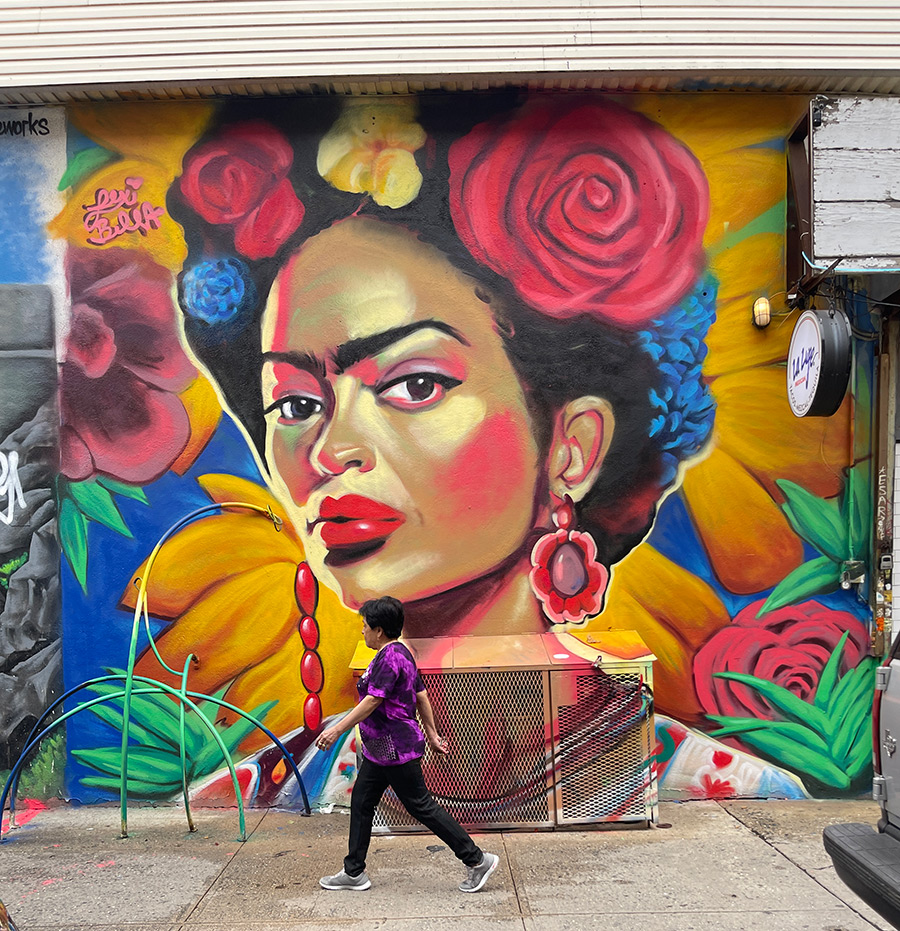The image showcases a striking mural painted on the wall of a building, likely located in Brooklyn. The mural, which could span up to two stories in height, portrays the iconic Mexican painter Frida Kahlo from the chest up. Frida, depicted with dark skin, has her black hair swept back into an elaborate updo adorned with an array of colorful flowers; a prominent red rose stands out among blue, yellow, and additional red flowers in her hair. Her signature thick eyebrows nearly meet in the middle, and she's adorned with heavy makeup including bright red lipstick. She maintains a stern expression as she gazes outward. The background of the mural features bright yellow flower petals set against a vivid blue backdrop, with red and yellow flowers adding further vibrancy. In the foreground, a woman with light skin, dark black hair, and a bright purple shirt, black pants, and gray shoes is seen walking by, her height reaching approximately to Frida's chin on the mural. The upper corners of the image capture parts of the building's wooden roof, while the lower corners display the cement sidewalk and painted poles. The mural’s vivid detailing and sheer scale make it a captivating urban art installation.